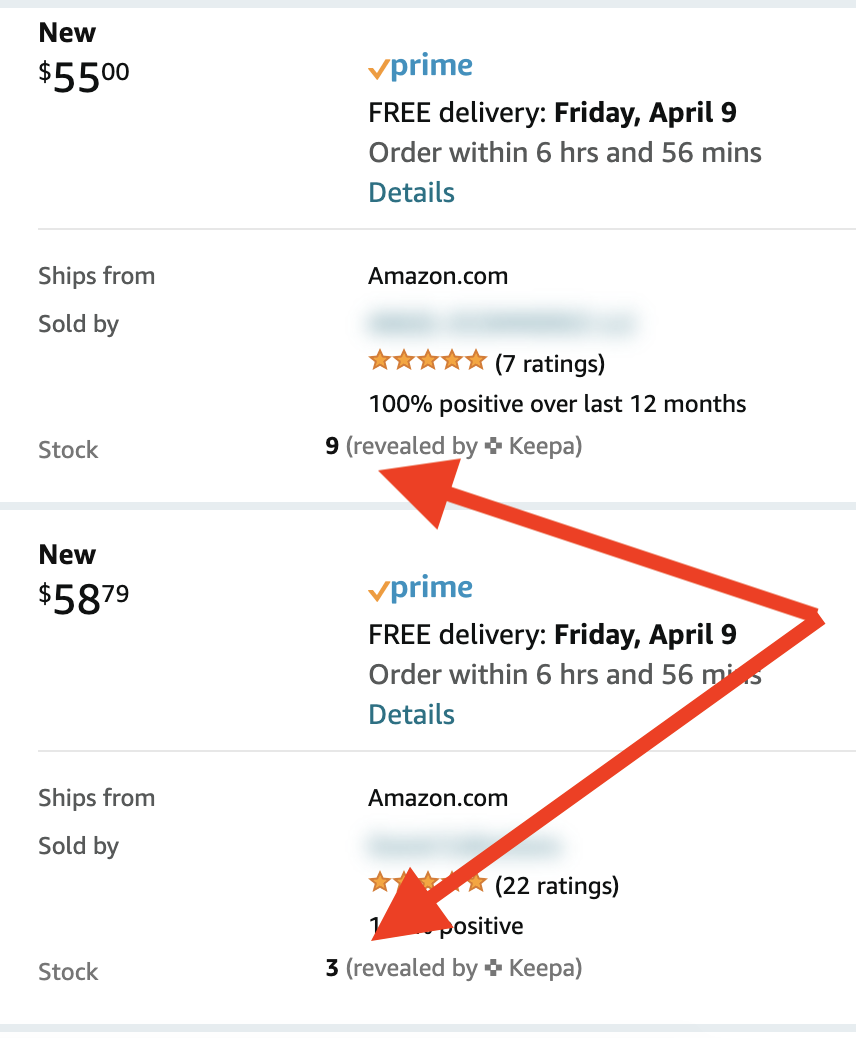In the provided image, the scene appears to be a screenshot from Amazon Prime displaying a list of items with their respective prices and delivery information. Although the actual items are not visible, the chart details are clearly present:

At the top, in bold black text, it shows: "New $55." To the right, it prominently displays "Prime" and "Free Delivery, Friday, April 9th" in bold. Below this, the text instructs, "Order within six hours and 56 minutes," followed by "Details."

Next, it mentions that the item "Ships from Amazon.com" and is "Sold by" a seller whose name is blurred out. Underneath, the listing features a rating of "Five stars with seven ratings" and indicates, "100% positive over the last 12 months." The availability is shown as "Nine revealed by Keepa," indicating there are nine items in stock.

A gray line separates this entry from the next one below it.

The subsequent listing states: "New $58.79," followed by "Prime," and the same delivery information: "Free Delivery, Friday, April 9th" and "Order within six hours and 56 minutes," with "Details" underneath.

Similar to the previous entry, this item is described as "Ships from Amazon" and "Sold by," with the seller's name also blurred out. This listing has received "Five stars with 22 ratings" and indicates that "Three" items are in stock, as revealed by Keepa. Red arrows point toward the stock levels of both listings: nine for the first item and three for the second item.

The image provides a detailed comparison of the two Amazon Prime listings, highlighting the differences in price, stock availability, and customer ratings.